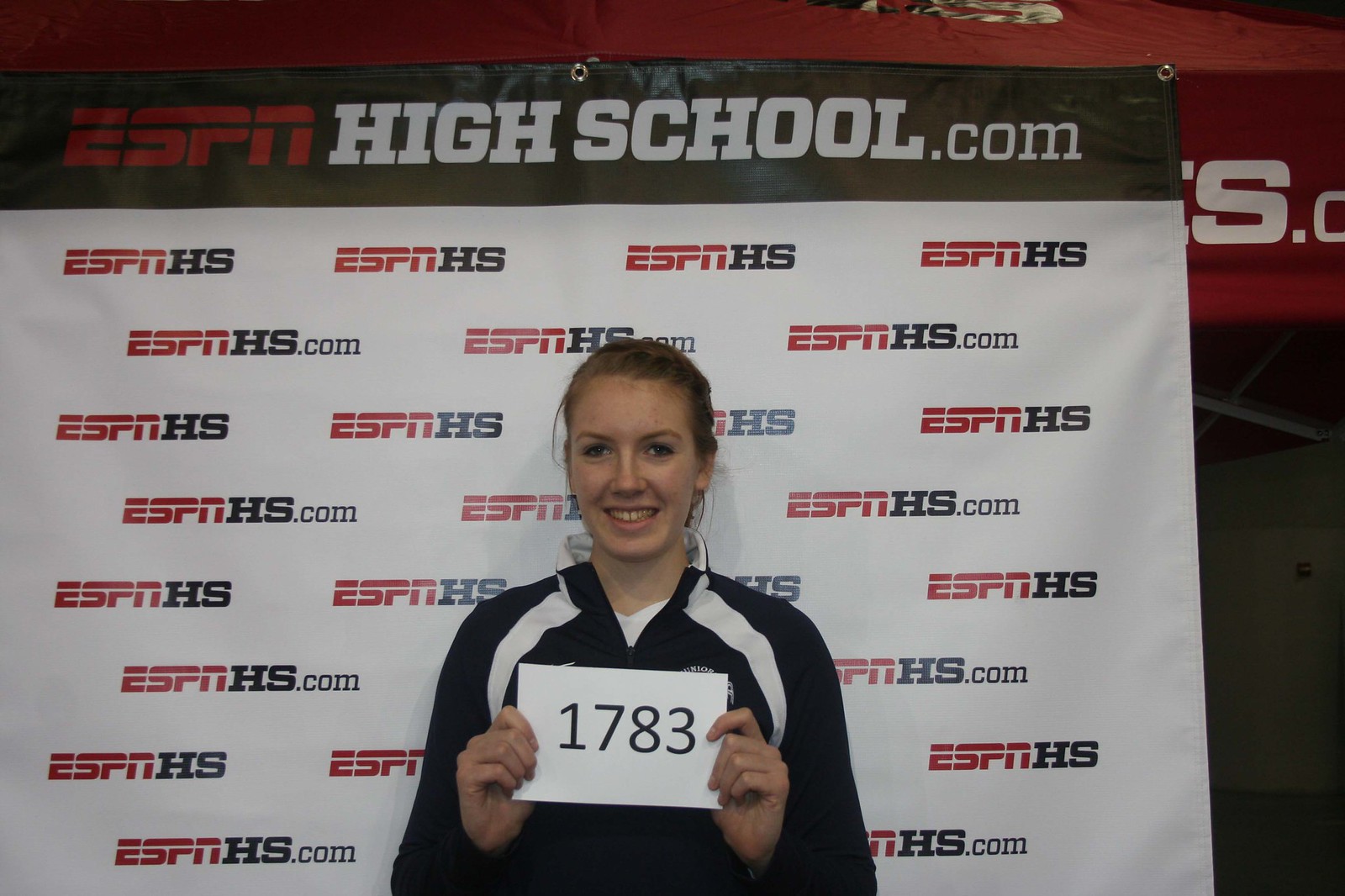A vibrant color photograph features a smiling teenage female athlete standing proudly in front of a white ESPNHighSchool.com banner, decorated with numerous repeating ESPNHS and ESPNHS.com logos. Her blond hair is neatly pulled back into a ponytail, accentuating her joyous expression. She is clothed in a dark blue, possibly black, long-sleeve shirt with distinctive white stripes running from the shoulders to under the arms. Clutched in her hands, she presents a white card prominently displaying the black numbers "1783." The banner behind her sports a black top bar with "ESPN" in striking red letters and "highschool.com" in white letters beneath it. The young athlete beams with happiness, embodying the spirited energy of a high school sports event promoted by ESPN High School.